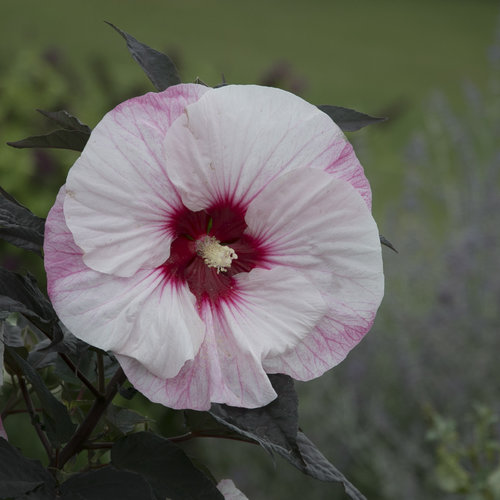This is a close-up photograph of a fully bloomed infucia flower in its natural environment, capturing its intricate details with remarkable clarity. The flower, which occupies the majority of the frame, showcases large, delicate white petals with pale pink tips. These tissue-like petals overlap in a circular pattern around the central pistil, which features a dark burgundy hue and pale cream-colored buds adorned with striations and veins. At the heart of the flower, the stamen and pollen are visible, exhibiting a mix of dark burgundy and beige colors. The flower is supported by a dark green stem with slender, pointed leaves, also dark green, that hang gracefully underneath. The background is artfully blurred, hinting at a garden or field with additional flora, including hints of purples and yellows amidst the green vegetation, ensuring the main focus remains on the exquisite bloom.